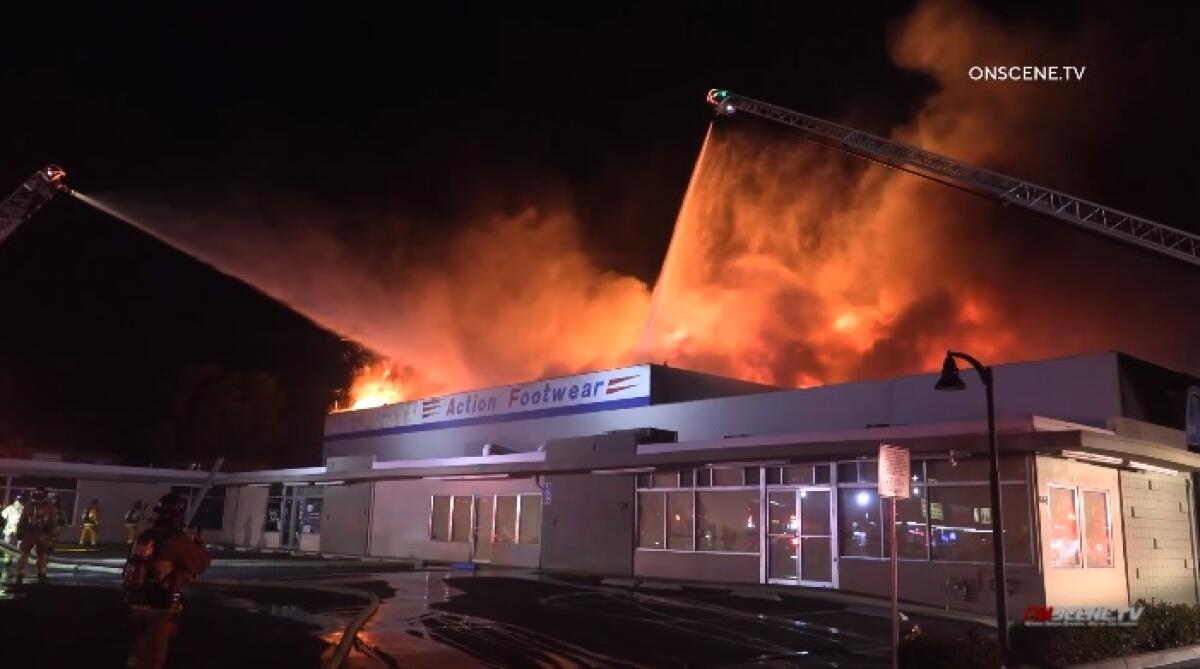This nighttime photograph captures a dramatic scene at a retail store engulfed in flames. The store, named Action Footwear, is a single-story, gray commercial building with its windows obscured by brown paper, indicating it was closed. The roof glows ominously with red, yellow, and orange flames, visible flaring out into the night. Firefighters are valiantly combating the blaze using ladder-mounted water hoses—one crane positioned to the right and another to the left, both directing streams of water towards the roof and the Action Footwear sign in blue and white font. Additional firefighters are poised on the ground, ready to breach the building to control the fire. In the lower right corner of the image, there's a label reading "ONSCENE.TV" in white, adding a sense of ongoing reportage to this intense emergency scene. The parking lot in front of the building is strewn with fire hoses and bustling with men in firefighting gear, illustrating the coordinated effort to extinguish the flames.